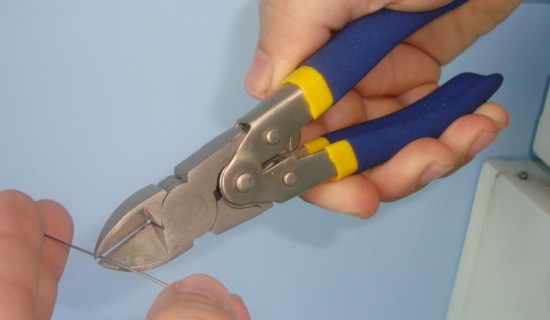This image captures a detailed scene of someone cutting a thin silver wire with a pair of substantial wire-cutting pliers. The individual, who has light Caucasian skin with slightly long and somewhat dirty nails, is using their right hand to grip the pliers. The pliers have bright blue handles with a yellow stripe near the top, leading to the dull silver cutting jaws. The hand holding the pliers extends downward from the upper right corner of the photograph, while the other hand, visible in the lower left corner, positions the wire for cutting. The background features a light blue wall and the edge of a white equipment piece, potentially a washing machine, with a visible screw. The scene is well-lit, casting a slight shadow behind the hand, emphasizing the meticulous action about to take place.